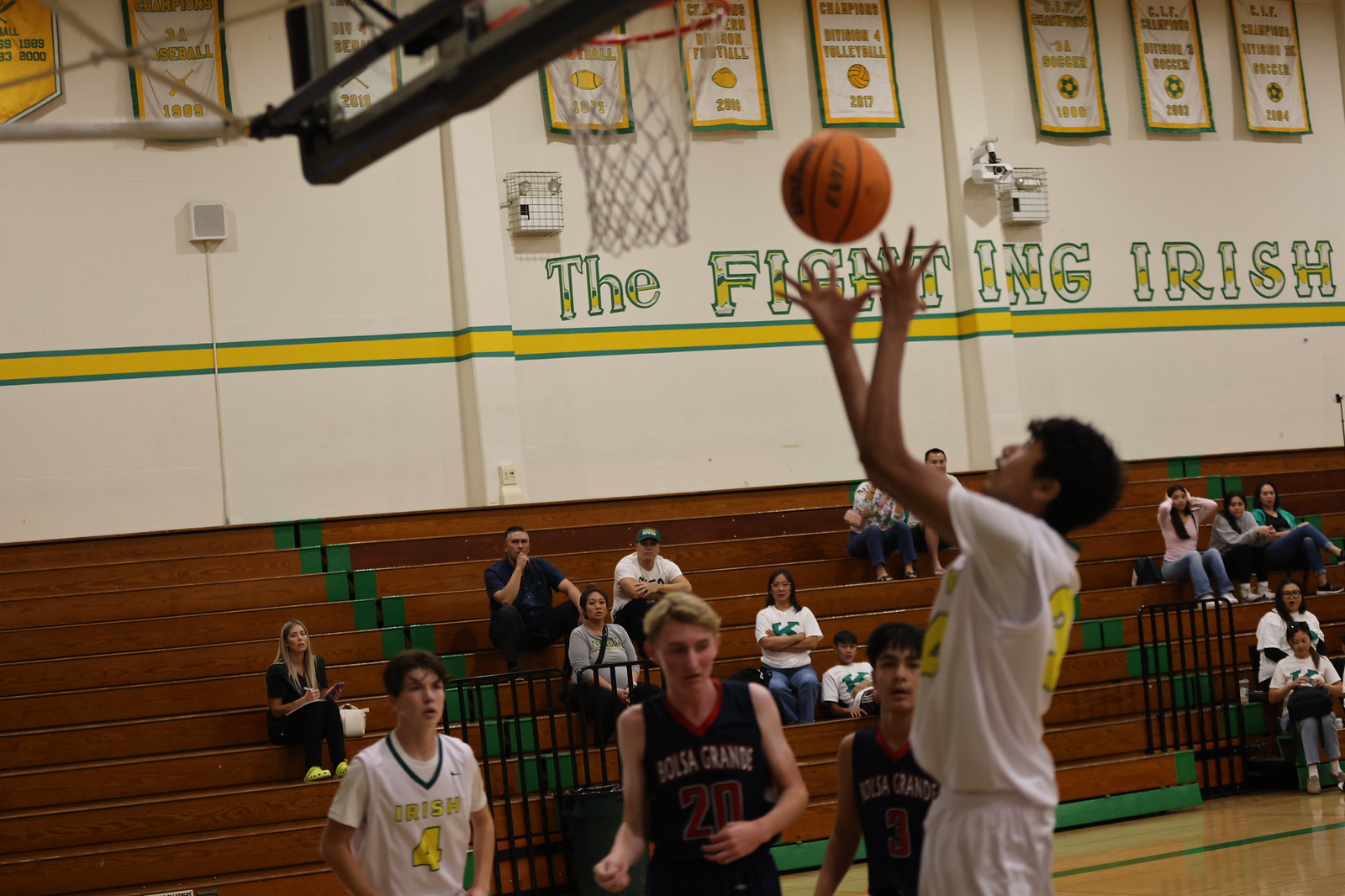In this photograph, a thrilling moment in a high school basketball game is captured. The scene is set in a gymnasium, where a teenage player from the Fighting Irish team is leaping into the air, the basketball having just left his hands in an attempt to score. Opposing him are two members of the Bolsa Grande team, with one player, number 20, positioned in front trying to block the shot, while another trails behind. On the court, two more Fighting Irish players can be seen, one of them wearing number four, while the number of the shooting player remains obscured.

The gymnasium provides a vibrant backdrop with its bleachers sparsely occupied by family members and fans. Above the bleachers, banners celebrate the team's achievements, and the words "The Fighting Irish" are prominently displayed. The photograph, captured from behind and slightly to the right of the basket, may appear amateur due to its angle, but it vividly conveys the action and spirit of the game.